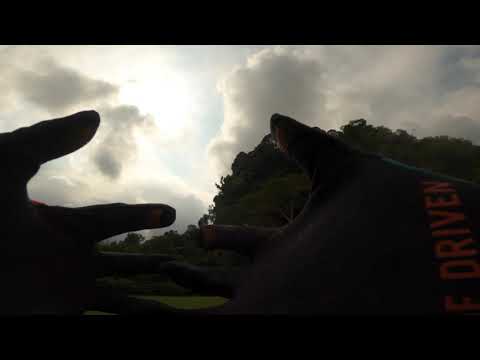This high-contrast photograph captures a pair of hands, prominently dark and splayed against a bright, cloud-filled sky. The left hand intrudes from the edge of the frame, with the thumb and index finger clearly visible while the other fingers fade into the shadowy background. Positioned on the right side, the other hand is faintly discernible, wearing a glove with the word "DRIVEN" (or "E-DRIVEN") inscribed on it. In front of the hands, a small hill, crowded with indistinct, shadowy tree leaves and foliage, further darkens the scene due to the intense sunlight. The backdrop features a bright, sunlit sky populated with puffy grayish clouds, with a black border occupying the top 12-15% of the image, adding to the overall dim ambiance.